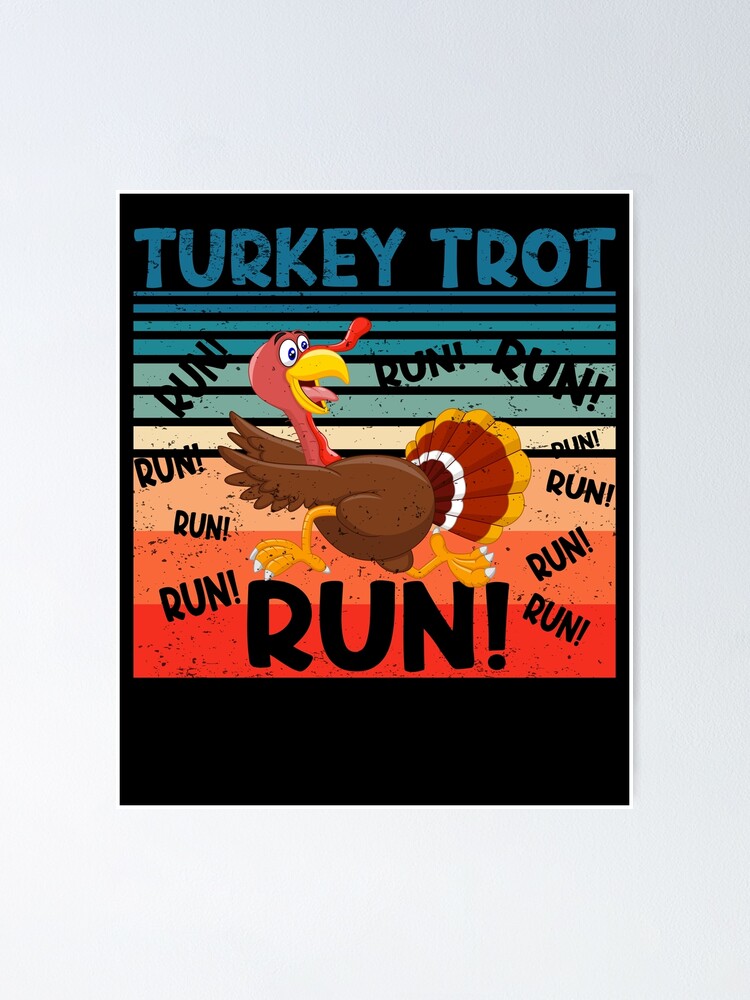The flyer advertising a fun running footrace, titled "Turkey Trot" in distressed blue lettering at the top, features a vibrant, cartoon turkey in mid-run across a black background. The turkey, with its red head and neck, brown body, and yellow feet, is depicted dashing to the left while glancing back to the right. Its colorful tail feathers are illustrated in shades of orange, white, and gold, which match its beak and feet. Adding dynamic motion, part of its face appears to flap in the wind. Surrounding the turkey are multiple iterations of the word "RUN!" in a circular pattern, accentuating the sense of movement and urgency. The background includes a sequence of peach, tan, and red rectangles at the bottom, which blend into a gradient of colors progressing from light red and orange to a darker teal and blue towards the top. Black lines run through the upper part of the image, enhancing the overall dynamic design of this lively and engaging poster.